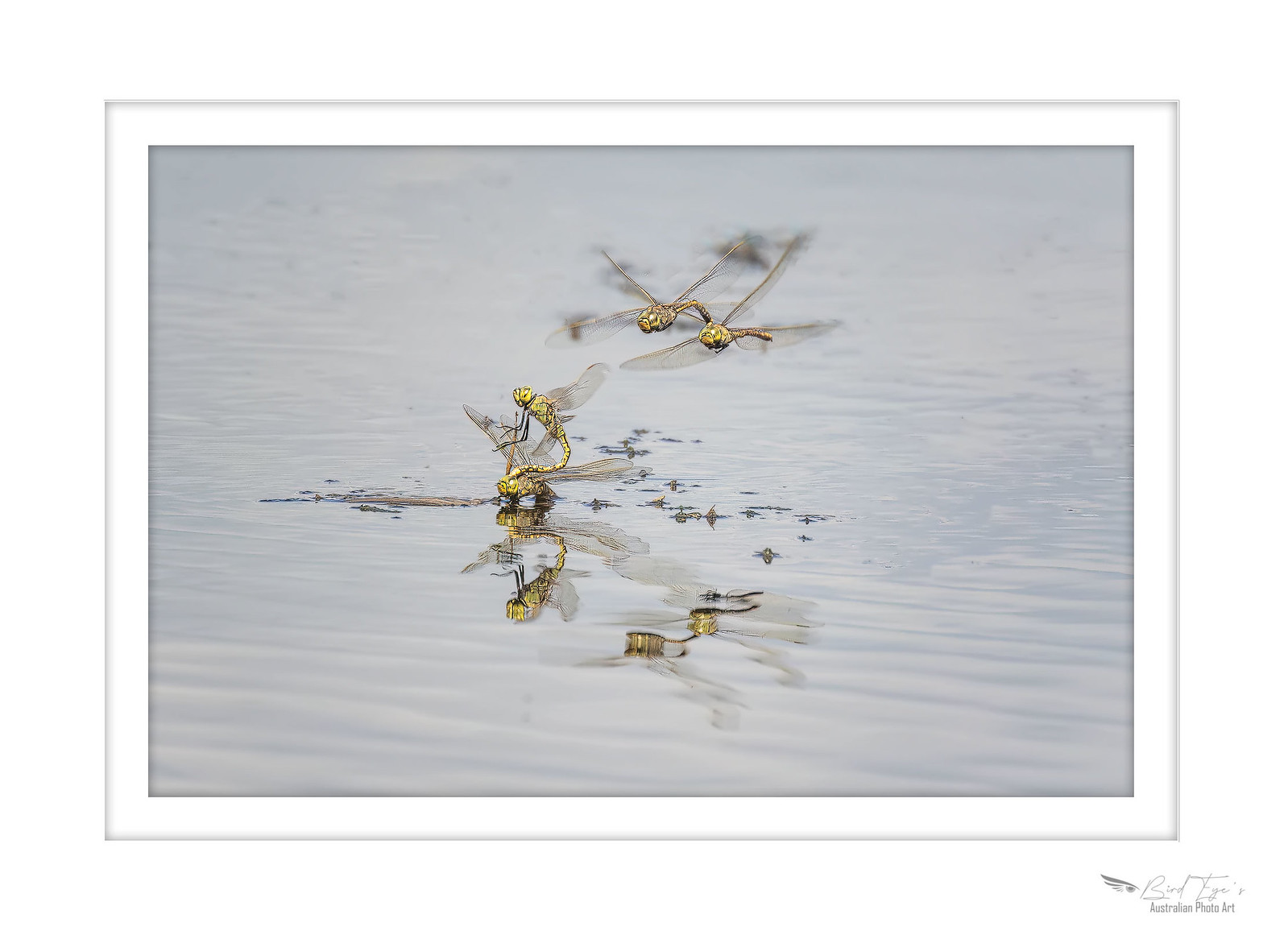This captivating image, presented within a white picture frame, depicts a serene scene of nature. The artwork, which appears to be either an altered photograph or a detailed painting, shows a body of water with subtle blue-gray hues. Running horizontally though slightly diagonally from left to right, fine lines enhance the effect, mimicking the gentle ripples of the water surface.

At the center, the main focus is on four dragonflies, strikingly colored in yellow and gold with black accents on their wings. Two of these vibrantly detailed dragonflies are depicted diving towards the water, creating tiny splashes and suggesting they might be feeding. Positioned just above them, the other two dragonflies hover gracefully in flight. Their reflections are cast clearly on the calm water below, giving the illusion of a larger gathering of dragonflies.

In the bottom right corner of the image, there is a faint signature, possibly reading "bird, tiger" along with the notation "Australian photo art," indicating the potential Australian origin of the artist. The image beautifully captures a moment of natural activity, emphasizing the dragonflies' interaction with the water and their lifelike reflections.